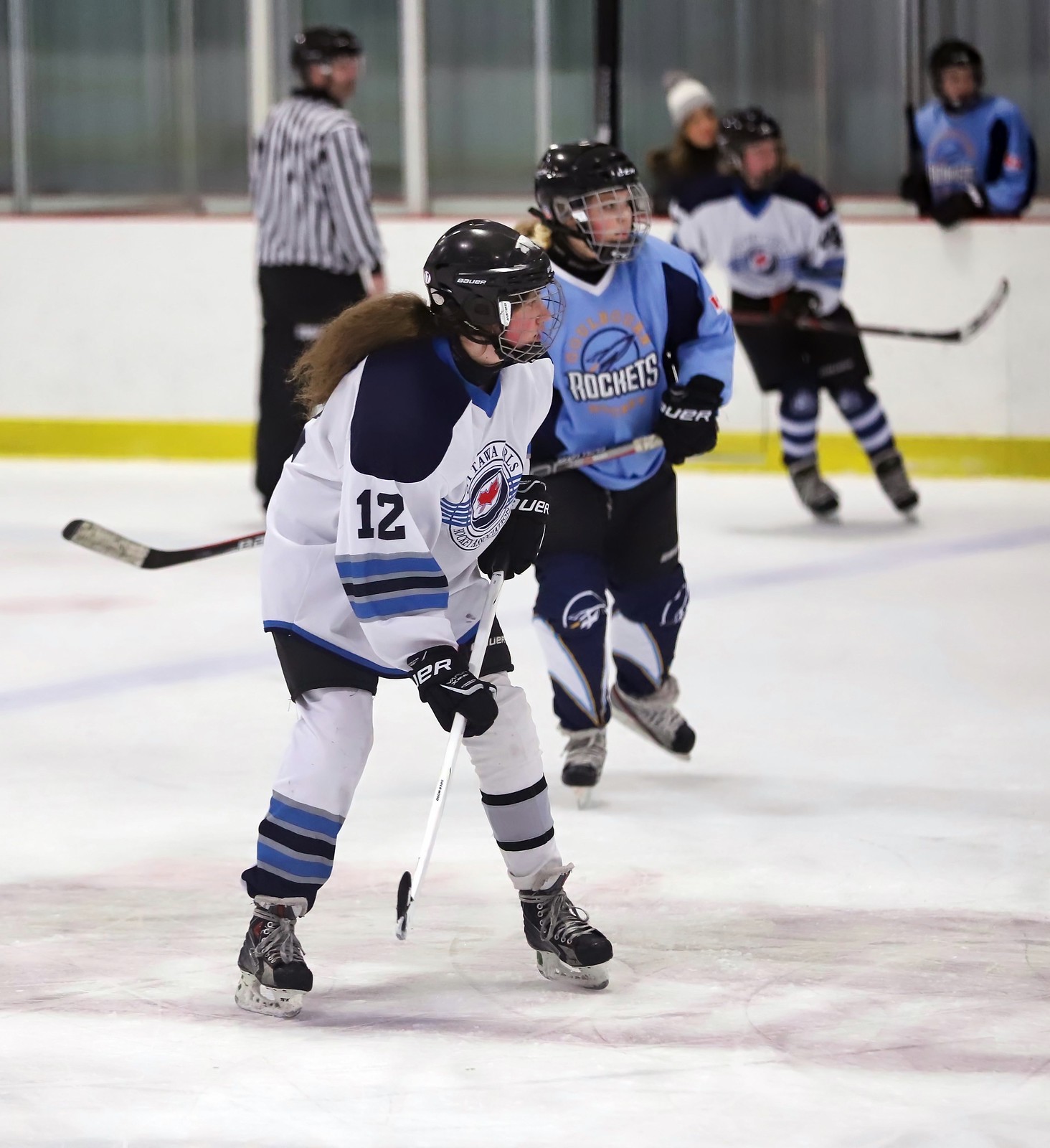This detailed photograph captures an intense moment in a women's ice hockey match featuring two teams. The team in white jerseys with navy blue details is opposed by the team in light blue jerseys with black accents, prominently displaying the name "Rockets" along with a rocket emblem within a circle. The central focus is on two main players in the foreground: the front player, number 12, donned in the white and navy jersey, wields a white stick and skates with long brunette hair tied back. She features blue stripes on one legging and gray and white stripes on the other. Close behind her is a player from the Rockets team, outfitted in a light blue jersey with a white v-neck, holding a black stick across her abdomen. Both players are framed by four additional figures in the image, including a referee in a striped shirt standing directly behind them. The background captures a blurred view of another player in a white uniform, another Rockets player partially obscured behind the wall, and a person in a dark top, likely a manager. The scene is set on the ice, encapsulating the dynamic and fast-paced nature of the sport.